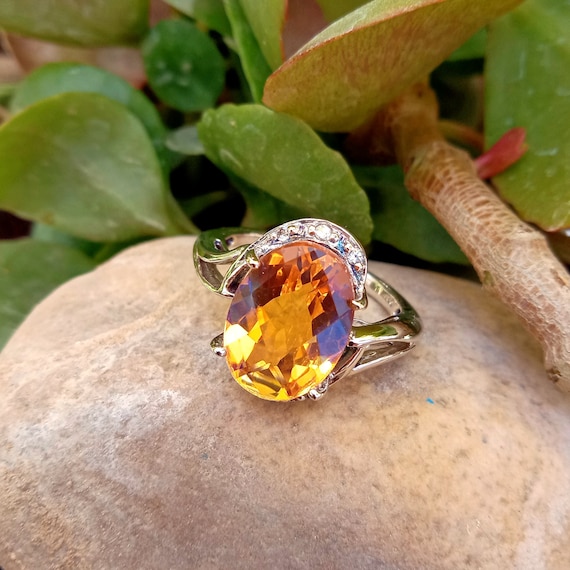The image showcases a silver ring adorned with a large oval gemstone that transitions from yellow at the base to blue and darker yellow hues towards the top. The gemstone is set in a silver, possibly white gold, setting and is further embellished with several small diamonds. The ring is elegantly perched atop a light brown to tan stone. Surrounding this stone are various green leaves, adding a natural backdrop to the outdoor scene. Adding to the intricate details, a thicker stick lies across the stone, creating a rustic aesthetic. The combination of the reflective gemstone, detailed ring setting, and natural elements highlights the serene and intricate beauty captured in this image.